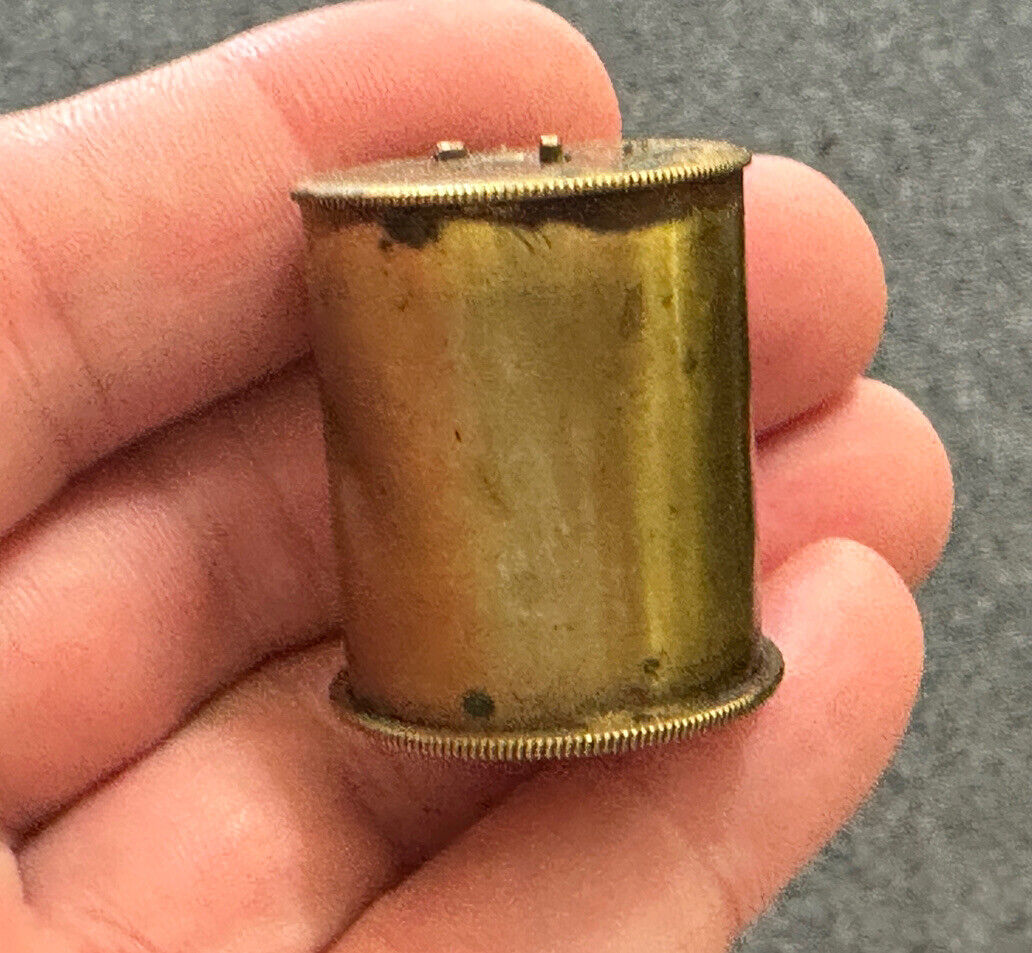The image is a very blurry and grainy close-up photo, likely taken with a cell phone, depicting a Caucasian man's hand holding a small, cylindrical, golden object. The object resembles a film roll or spool and features indented, ribbed details around its top and bottom edges, similar to a coin's serrations. The spool is notably tarnished and distressed in some areas, particularly around its top and bottom. Given the perspective and focus on the fingers, the object's exact purpose is unclear, though it fits comfortably within the fingers of the person's hand. The backdrop of the image is a gray, pixelated surface that may be some type of rug, carpeting, or possibly pavement.